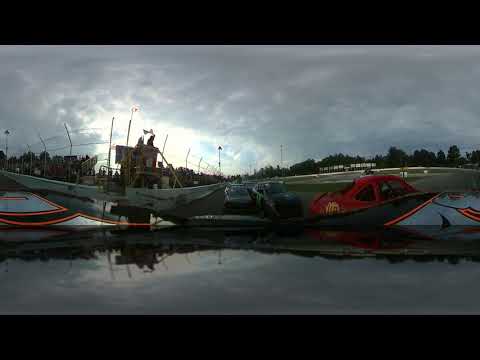The image captures a vibrant and dynamic racing scene, likely set during the daytime at an amateur stock car racing event. Taken from a wide-angle or fisheye lens mounted on the rear of a black race car, the photo showcases the intensity of the race. The action unfolds on an oval racetrack, surrounded by a high white barrier wall that matches the height of the cars. Behind the featured black car, the track is teeming with competitors, including a prominent red car with yellow writing to the right and a series of black cars with various markings further behind.

The backdrop reveals a grandstand filled with spectators, adding to the lively atmosphere. The center of the track boasts a patch of green grass encircled by the tarmac. Though the sky is predominantly gray and overcast with clouds hinting at rain, patches of blue sky peek through on the left side, where a bright white glow from the sun illuminates the scene. This snapshot captures a crucial moment, possibly just past the finish line, as someone waves the checkered flag from the stands, marking the culmination of the race.